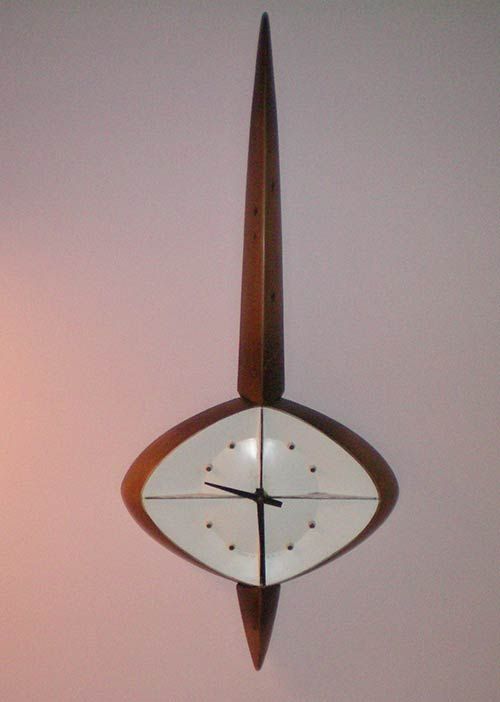This image features a retro wall clock, evocative of designs from the 1950s or 1960s, or perhaps a reproduction of that era. The clock is uniquely shaped, akin to a smushed square or an oblong diamond with rounded edges, set against an off-white gray wall. The clock's frame is crafted from brown wood, giving it a warm, vintage feel. The face of the clock is predominantly white, divided into four quadrants by a simple cross. Instead of traditional numbers, the 12, 3, 6, and 9 positions are marked by lines, while the other hours are denoted by minimalistic dots. The clock's hands are black. At the 12 o'clock position, there is a distinct elongated wooden spear-like ornament that extends vertically, mirroring a smaller arrowhead-shaped piece at the 6 o'clock position. The time displayed on the clock is 6:47.